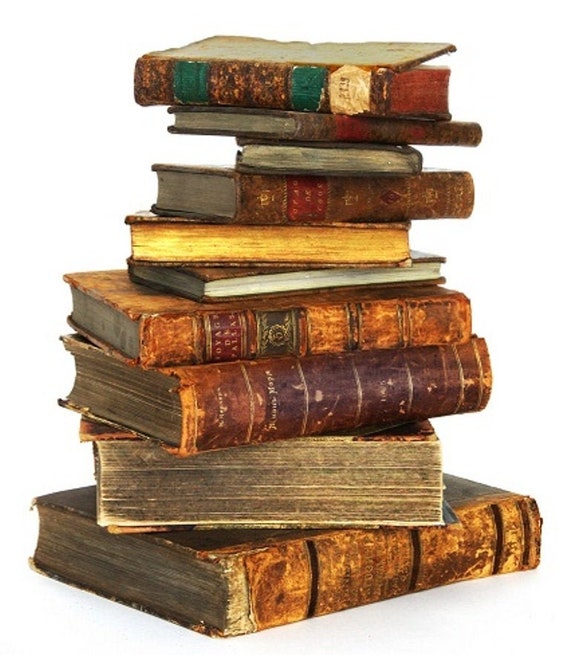The image features a photograph of an unevenly stacked pile of ten antique books, arranged on their sides. The books exhibit significant signs of wear, with ragged, faded covers and bindings, and pages that range from cream to yellow hues, with darker patches visible in places. The largest book sits at the bottom of the stack, turned at an angle, while subsequent books are positioned at alternating angles, revealing different parts of each. Notably, the third and fourth books from the bottom have visible spines; one displays a brown spine with red lettering that appears to read "Voyage to something," and the other features a brown and gold spine with indistinct gold lettering. As the stack progresses upward, the books gradually diminish in size, with the smallest and thinnest book perched at the top. The overall stack is haphazard, jutting out at various points, with no alignment or symmetry. The photograph is set against a plain white background, highlighting the age, collectible nature, and worn condition of the books.